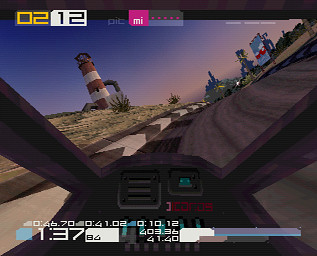This is a detailed screenshot from a video game, capturing a tense moment on a racetrack. The player's vehicle is shown navigating the track, flanked by a striking red and white striped lighthouse on the left side. Alongside the road run black and white directional arrows, guiding the way. Displayed at the top of the screen is "O2-12," along with "MI" for miles, distinctly highlighted in pink with dots beside it. The bottom of the screen features the numbers "137" along with several other indicators. The cockpit view of the vehicle reveals a panoramic window at the top and two side windows, providing a clear view of the surroundings. To the right, a billboard comes into view, depicting a cityscape in the background, adding to the immersive racing experience.